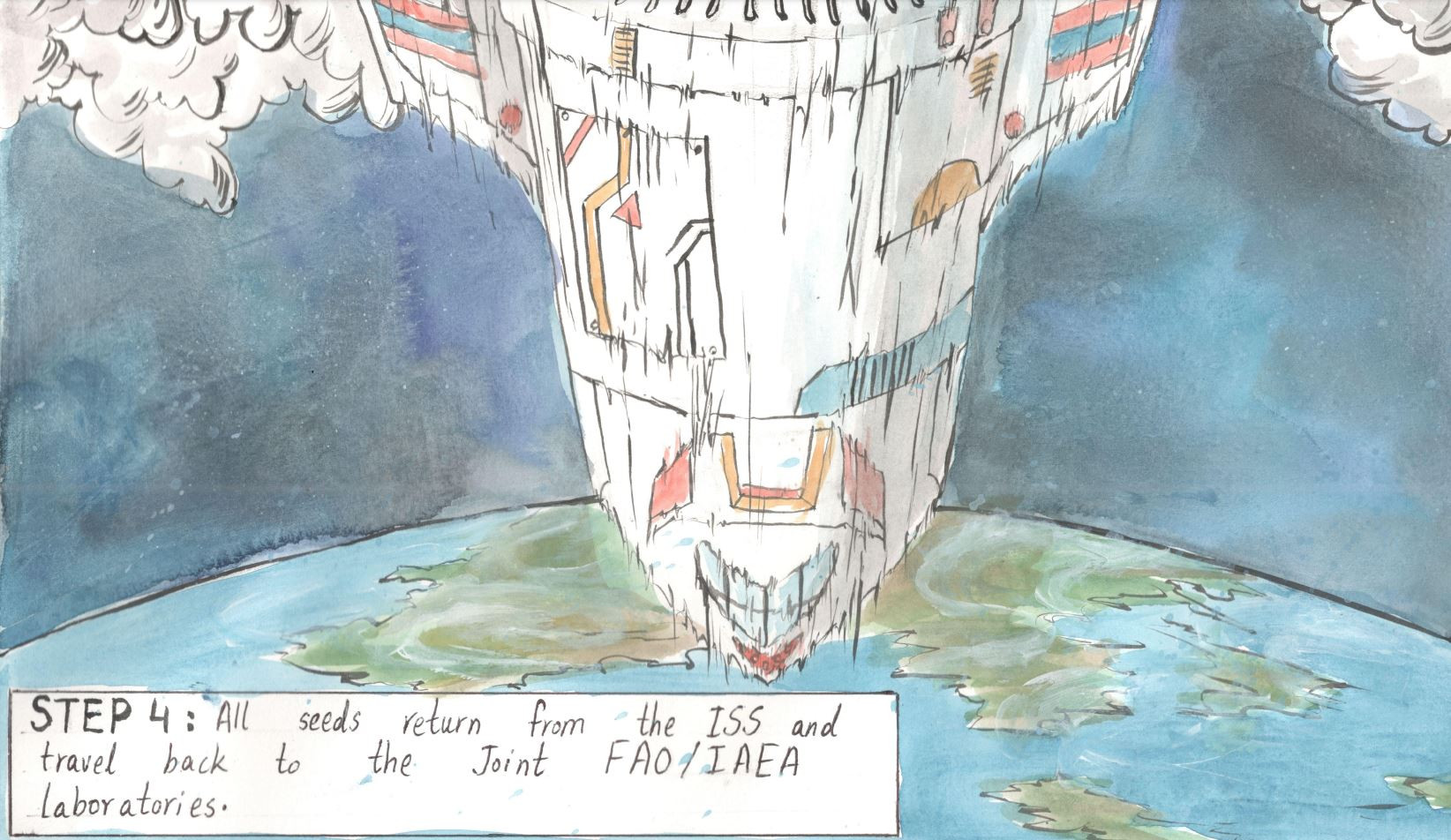The image depicts a drawn illustration reminiscent of a child's artwork or a chalk drawing. Dominating the center is a white rocket ship descending toward Earth, exemplifying a triangular cockpit with blue windows. Both the upper left and right quadrants feature stylized puffs of smoke or clouds, potentially from the rocket's jet engines, set against a dark, mystical backdrop of blue and purple space. The Earth occupies the bottom quarter, vividly showcasing blue waters and green and brown landmasses. A long rectangular space in the bottom left corner contains the text: "Step 4: All seeds return from the ISS and travel back to the joint FAO/IAEA laboratories." The spacecraft, partly visible with sections repeating cuts off including its wings, is adorned with blue, pink, and yellow markings, possibly representing a flag. The overall image intertwines the whimsy of outer space with the detail of a mission, perhaps illustrating the return journey from the International Space Station.